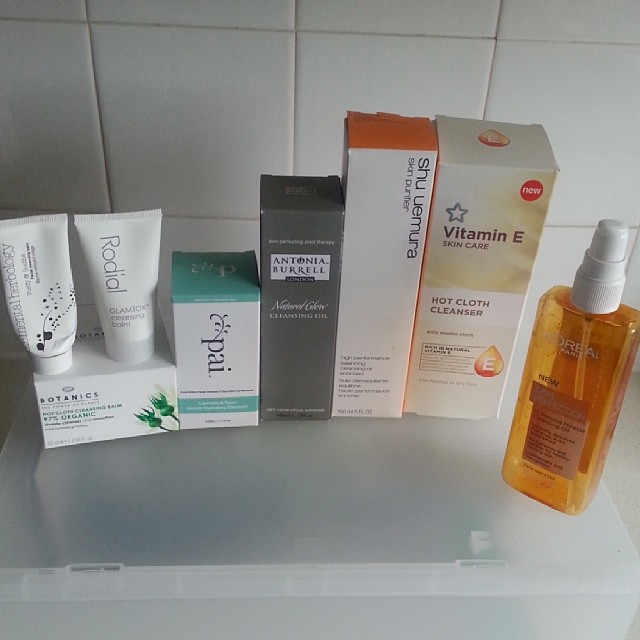The image depicts a bathroom shelf or storage box made of semi-translucent plastic, possibly with a lid, placed against a background of white tiled wall. On top of this storage unit, several personal care items are arranged. To the right, there is a clear, square-shaped plastic bottle containing amber-colored liquid, labeled with "L'Oreal" and fitted with a white pump dispenser. Beside this bottle, there is a box with a golden top and white lower half, labeled with "Vitamin E." Next to it, a white box with an orange top reads "Shu Uemura Skin Purifier." Following this is a completely gray box with a white label that says "Antonio Purrell." Adjacent to it, there is a shorter white box with a blue top potentially labeled "Dial." Finally, a white box holds two upright tubes of skin cream, both in white packaging. The arrangement of these items suggests a well-organized personal care routine.